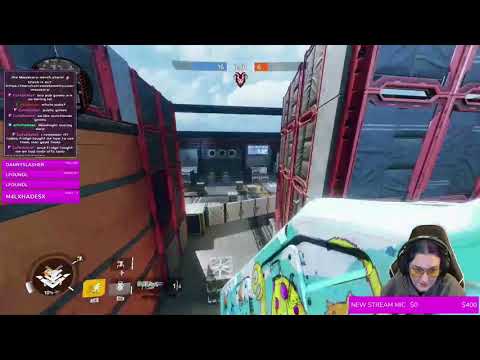The image is a wide rectangular scene from a video game with black borders on the top and bottom, giving it a letterbox appearance. The game’s setting appears to be an outdoor area between buildings or structures. In the center of the scene, there is an exit visible between two structures. The structure on the left is primarily light brown with dark gray or black borders, and behind it is a darker building featuring red borders. On the right side, there is another building that is gray or black, also with red borders. The background reveals more structures and a blue sky.

In the bottom right corner of the image, a woman with glasses and headphones is seated on a chair, seemingly playing the game, her attention fixed on a computer. She appears superimposed onto the game scene, giving a cut-out effect. Dressed in gray with black headphones, she has dark hair. Below her, there's a strip of fuchsia-colored text, though the content is too small to decipher. The overlay includes additional writing in fuchsia and black, likely messages from social media, situated in the upper left corner. Behind the woman, her surroundings suggest a cubicle or office space, characterized by dark brown and gray tones that fade into shadows, and decorated with bright, storybook-like characters, including yellow and polka-dot figures. Despite additional cubicles in the background, no other people are visible.